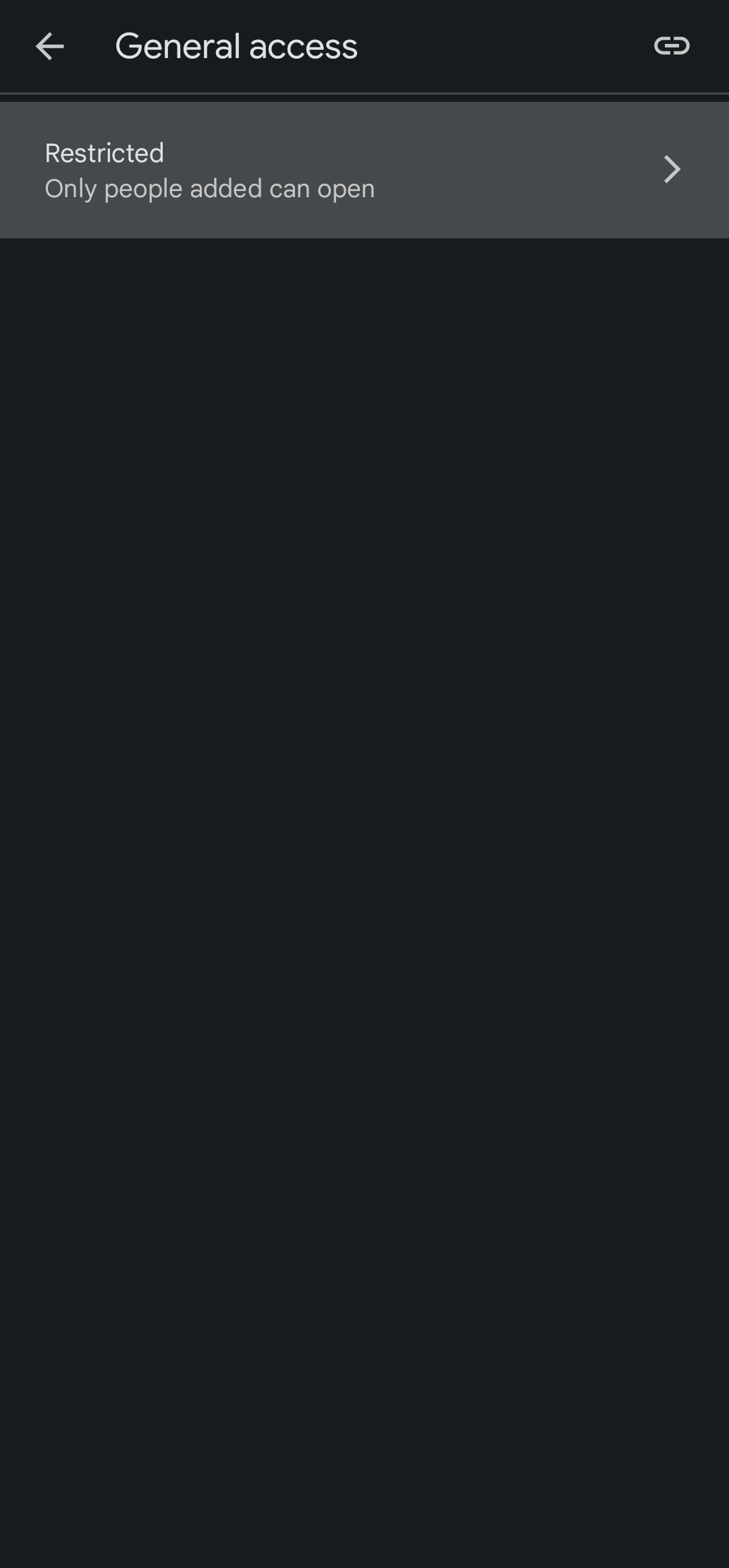The image depicts a predominantly black screen with a gray strip occupying the top third of the frame. Within this gray strip, a message in white text reads, "Restricted: Only people added can open." Above this strip, another label says "General access" in white font, accompanied by a white arrow pointing to the right. Adjacent to this text is a white paper clip icon. 

In the restricted area, the phrase "Only people added can open" reappears, this time accompanied by a white arrow pointing right. The rest of the screen remains entirely black, indicating that access is limited to specific users. There are no visible options suggesting recourse for those who believe they should have access, aside from the right-pointing arrow that might lead to additional options if clicked. Overall, the screen conveys that access to the content is strictly controlled, requiring explicit addition to the list of authorized users to view the material or information behind this restriction.